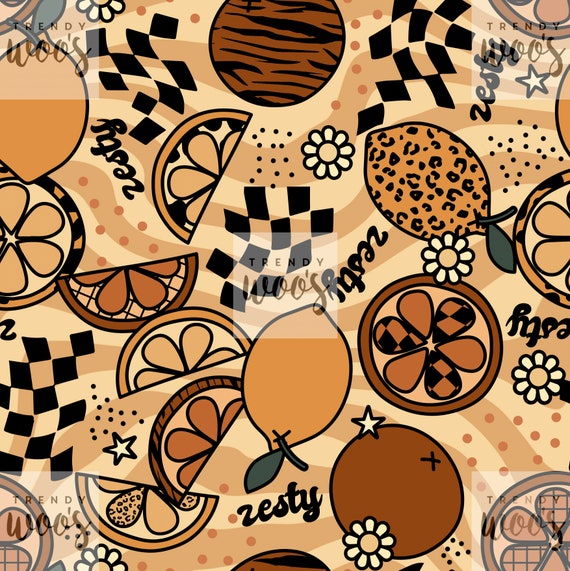This is an intricate brown, beige, and black drawing featuring various fruits and floral elements. Central to the artwork is a tan-colored lemon with a black leaf, highlighted repeatedly with the word "Zesty" written in different handwritings. Surrounding the lemon, the image showcases a mix of half circles and full circles filled with black checkerboard patterns and dark and light brown designs. Tiny, detailed elements, such as beige-centered off-white flowers outlined in black, and scattered black dots and stars add to the complexity. The drawing is subtly branded with the phrase "Trendy Woos" in the lower-left corner and repeated at every corner of the image. This artistic background blends both cartoonish and detailed elements, creating a visually stimulating composition.